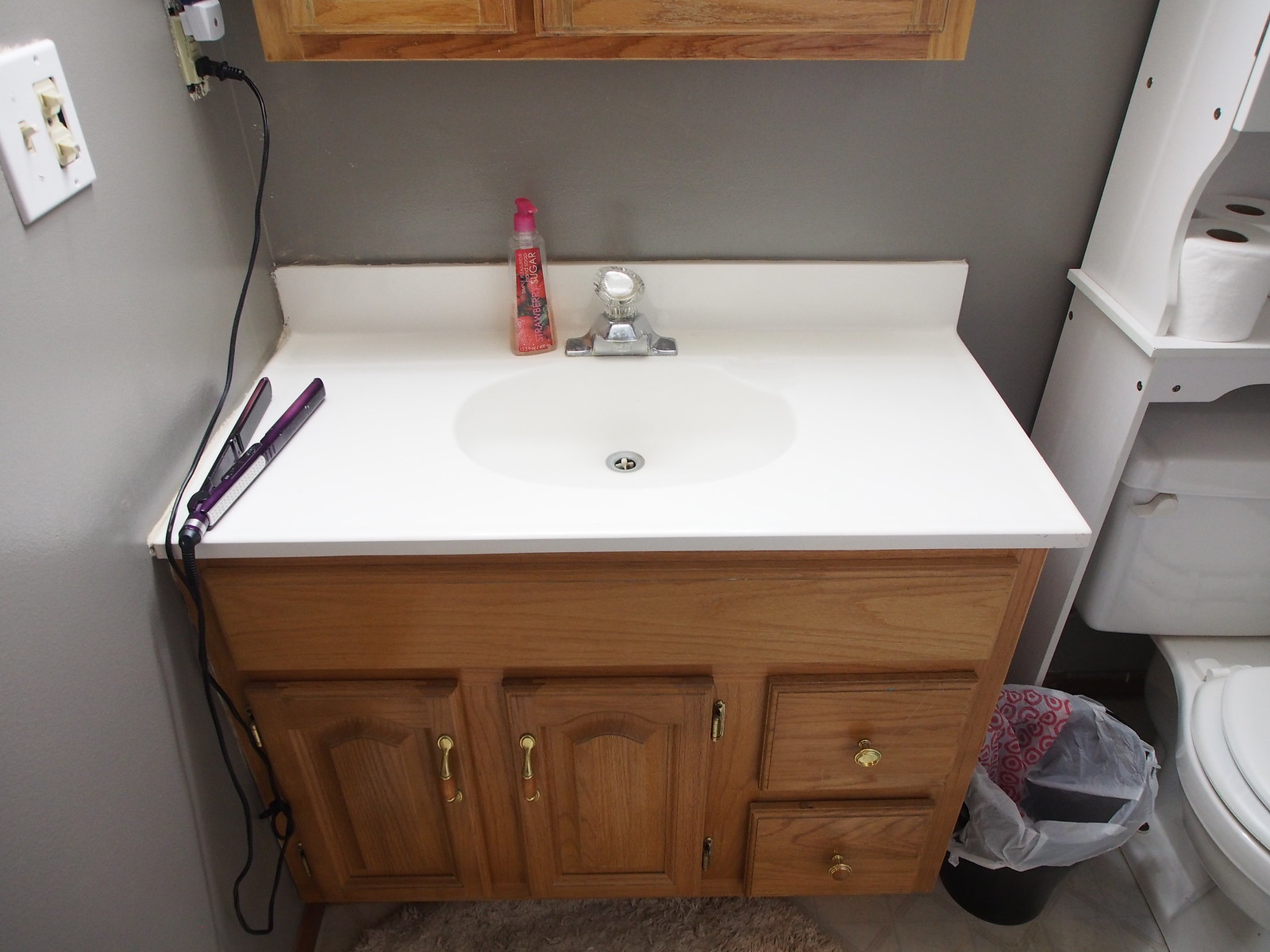The image depicts a typical American bathroom with a standard white toilet positioned centrally. Above the toilet tank, there is a white shelving unit extending approximately 5 to 6 feet high, featuring multiple tiers. The first shelf above the toilet tank holds a couple of white toilet paper rolls. The shelf above it is partially visible, with its contents cut off by the right edge of the photo. 

To the immediate left of the toilet is a black garbage can, which uses a repurposed Target shopping bag as a liner. Further to the left stands the bathroom sink and counter. The cabinetry beneath the sink is constructed from light, oak-colored wood, featuring drawers and cabinet doors. The sink itself is made of white stone, complemented by a chrome, single-handled faucet. A black curling iron rests on the countertop next to a bottle of red hand soap. 

The walls of the bathroom are painted in a gray hue, which matches the gray floor tiles. On the floor, there is a green rug mat, adding a splash of color to the otherwise neutral palette. Above the sink is a matching medicine cabinet, also in light oak, completing the coordinated look of the bathroom.